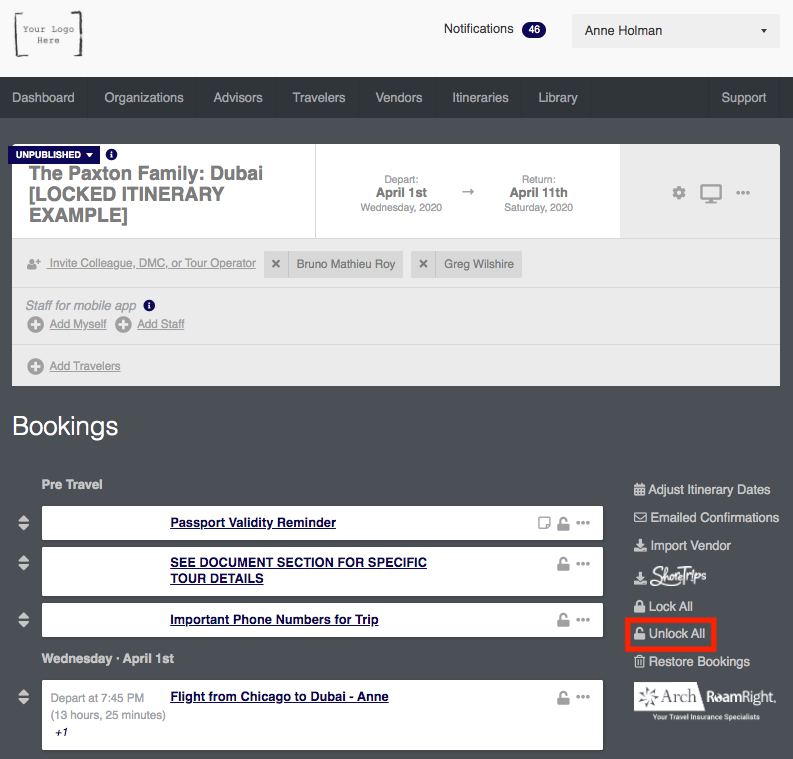**Detailed Caption:**

The image presents a sophisticated dashboard interface designed for travel management. The top of the interface includes tabs labeled "Dashboard," "Organizations," "Advisors," "Travelers," "Vendors," "Itineraries," and "Library Support." To the right, there's a circle indicating that Windows is unpublished within this environment.

Prominently displayed is an itinerary for the Paxton family's trip to Dubai, marked as a locked itinerary example. The journey is scheduled to depart on Wednesday, April 1st, 2020, and return on Saturday, April 11th, 2020. 

Key functions and features are visible, including icons for gear settings, screen adjustments, and inviting colleagues such as deans, CEOs, tour operators, and specific individuals named Bruno, Matthew, Roy, Greg Wilshere, and staff members. Options are available to add oneself, add staff, and add travelers.

Further elements include sections for bookings, pre-travel preparations, passport validity reminders, and a document section for specific tour details and important phone numbers. On Wednesday, April 1st, the flight departs from Trikook to Dubai, lasting 13 hours and 25 minutes.

To the right of the itinerary details are options for "Adjusted Itineraries," "Email Confirmation," "Import Vendor," "Lock All," and "Unlock All," with "Unlock All" highlighted by a red square.

There is also a prompt to "Restart Bookings." Some textual elements appear in a template style, with placeholders and marine green writing against a gray background, adding a structured but unfinished feel to some sections of the page.